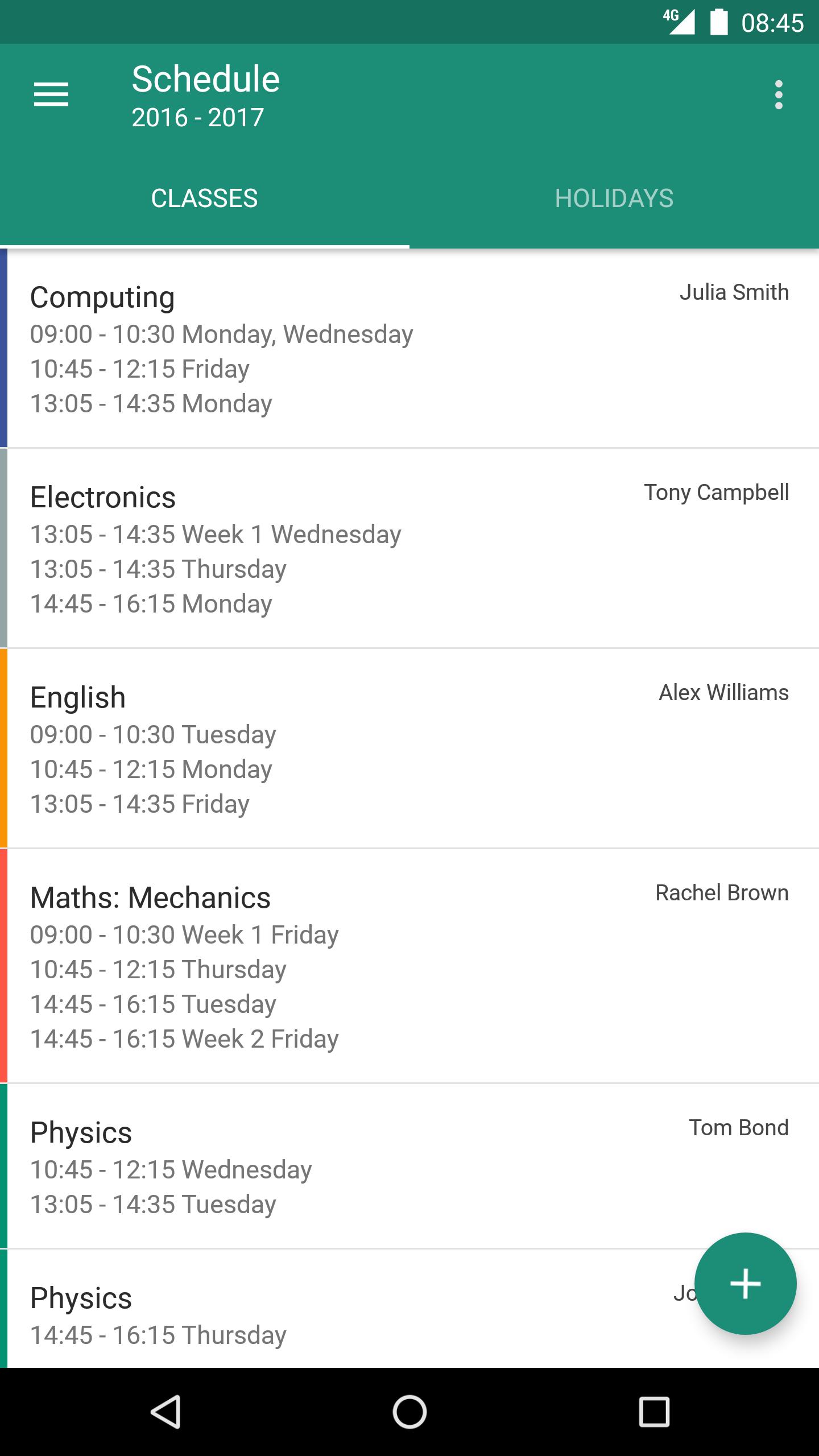**Screenshot Details of a Cell Phone Displaying a Class Schedule:**

The screenshot captures a cell phone screen at 8:45, though it is unclear whether it is AM or PM. The battery icon indicates a full charge and the phone is connected to a 4G network with full signal strength. At the top left corner of the screen, there is a three-line menu icon, suggesting a drop-down menu. On the right side, three vertical dots hint at another menu option.

Below the top menu bar, the screen displays the text "Scheduled 2016-2017." This is followed by two tabs: "Classes," which is currently highlighted, and "Holidays," which is not selected. 

The main content shows a detailed schedule of classes:

1. **Computing:**
   - Monday and Wednesday: 09:00 - 10:30 with Julia Smith
   - Friday: 10:45 - 12:15
   - Monday: 13:05 - 14:35

2. **Electronics:**
   - Wednesday (Week 1): 13:05 - 14:35 with Tony Campbell
   - Thursday: 13:05 - 14:35
   - Monday: 14:45 - 16:15

3. **English:**
   - Tuesday: 09:00 - 10:30 with Alex Williams
   - Monday: 10:45 - 12:15
   - Friday: 13:05 - 14:35

4. **Mathematics - Math Mechanics:** 
   - Details for this class are not fully provided.

5. **Physics:**
   - With Tom Bond and another instructor whose name is not specified. The detailed timing for these classes is not clearly mentioned.

This comprehensive schedule aims to meet the academic needs of the user, ensuring all classes and timings are well-documented for efficient time management.